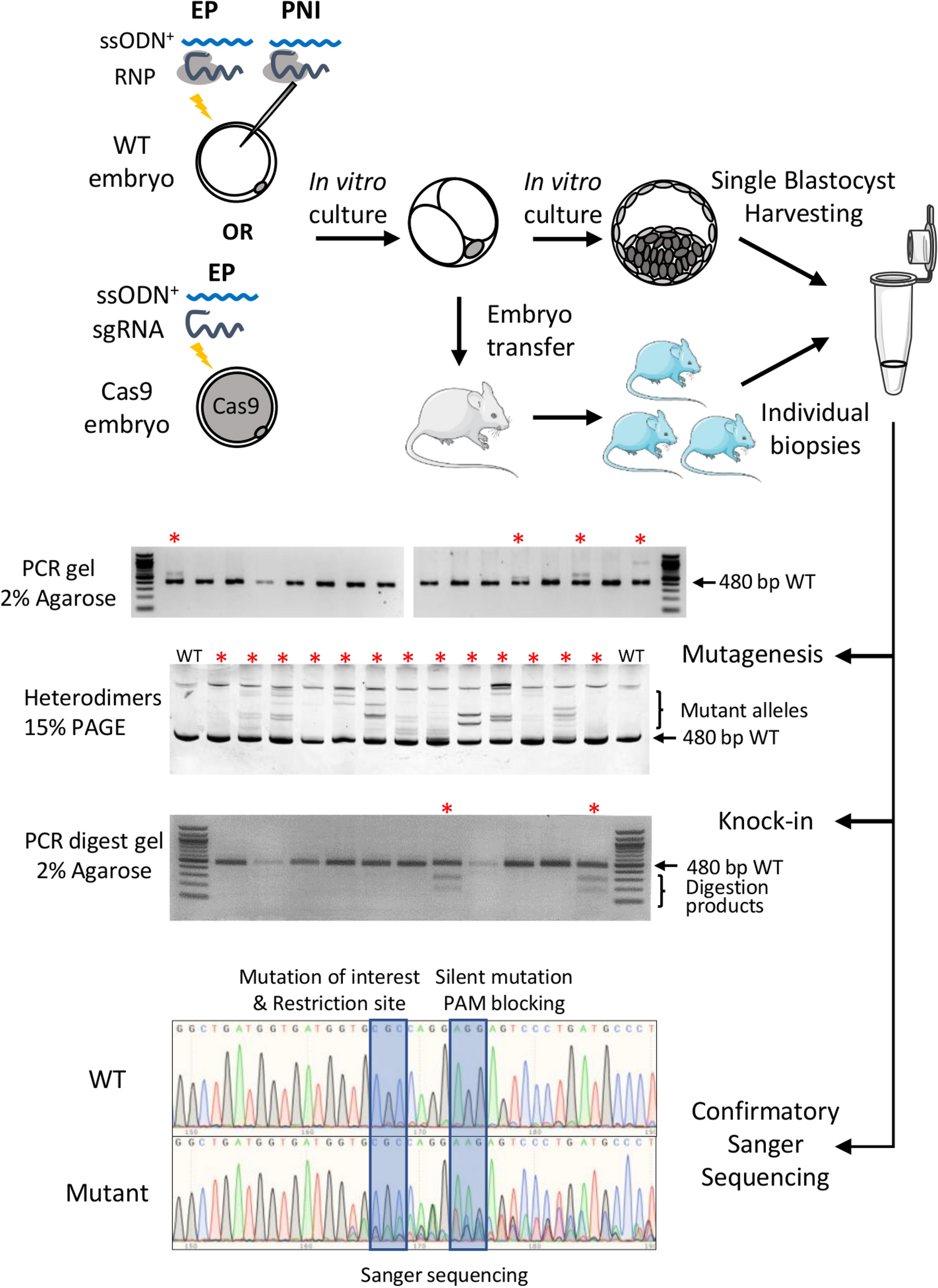The infographic details the complex process of in vitro fertilization and genetic modification in mice, from conception to the analysis of genetic mutations. At the top, two sequences labeled 'EP' and 'PNI' align with 'SSODN' and 'RNP' near blue squiggly lines, leading to 'WT embryo.' It shows a needle injecting something labeled 'embryo,' alongside another parallel process involving 'CAS9 embryo' and 'EP,' 'SSODN,' 'sdRNA.' Both pathways converge into a circle marked 'in vitro culture,' depicting a fertilized egg and cells at various stages. An arrow labeled 'embryo transfer' points to a mouse, and images of small mice and individual biopsies follow, indicating successive developmental steps.

Subsequent sections transition into genetic analysis. The 'PCR gel 2% agarose' reveals bands marked with red asterisks indicating significant markers underlined with '480 bp WT' and 'mutagenesis mutant alleles 480 BP WT.' 'Heterodimers 15% PAGE' indicates further data points with red asterisks. A 'PCR digest gel 2% agarose' segment is noted for 'knock-in' sequences with two indicating markers. 

Finally, a graph shows incidence rates labeled 'WT' and 'mutant,' depicted with distinct colored humps. 'Sanger sequencing' is denoted, highlighting areas of 'mutation of interest' and 'restriction sites,' accompanied by confirmatory genetic sequences GGCTGATGG, underscoring the DNA analysis aspect.

Overall, the infographic intricately maps from in vitro fertilization and genetic engineering in mice to the detailed stages of genetic testing.